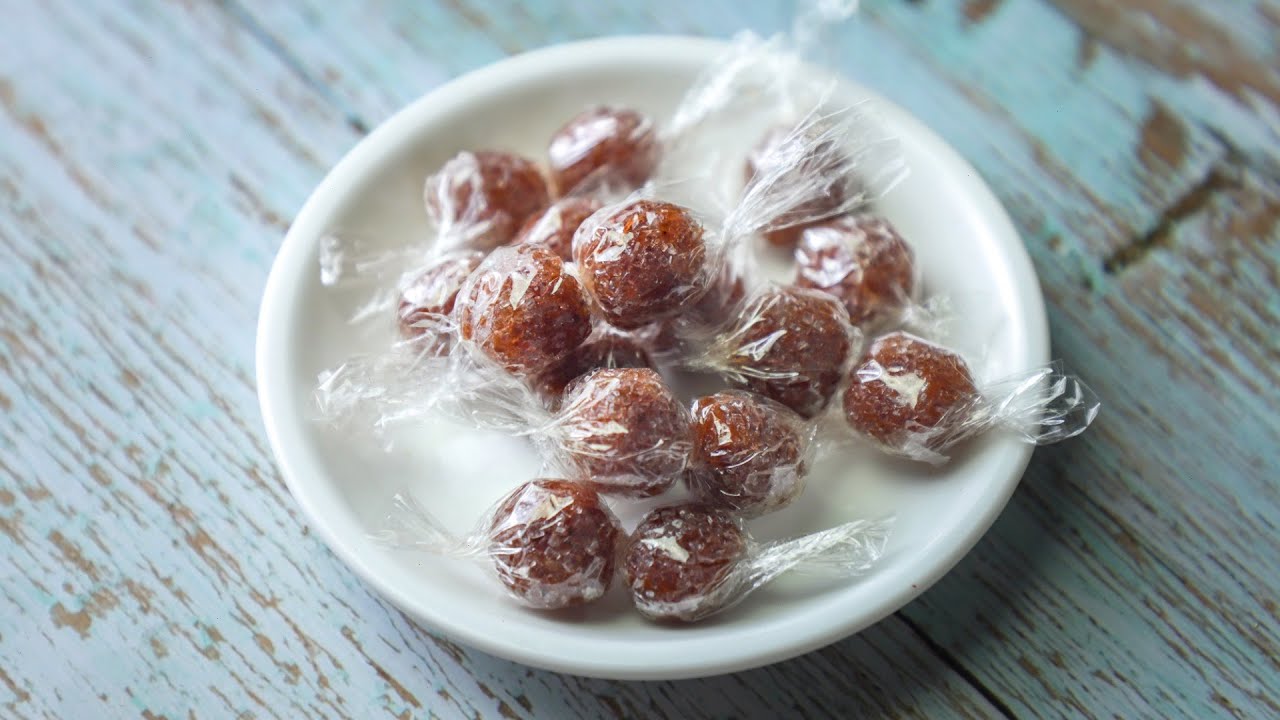The rectangular image features an aged, weathered wooden table painted in light blue with many brown scratches and chips showing through the faded paint. Centered prominently on this rustic surface is a small, white dish adorned with 10 to 15 individually wrapped, round brown candies. These candies, reminiscent in color to root beer barrels but distinctly spherical, are encased in clear cellophane with twisted ends. The arrangement in the dish appears slightly chaotic, with some candies stacked on top of each other, adding to the casual charm of the scene. The photo is taken from a slight above angle, emphasizing the textural contrast between the smooth, glossy wrappers and the rough, distressed wood beneath.